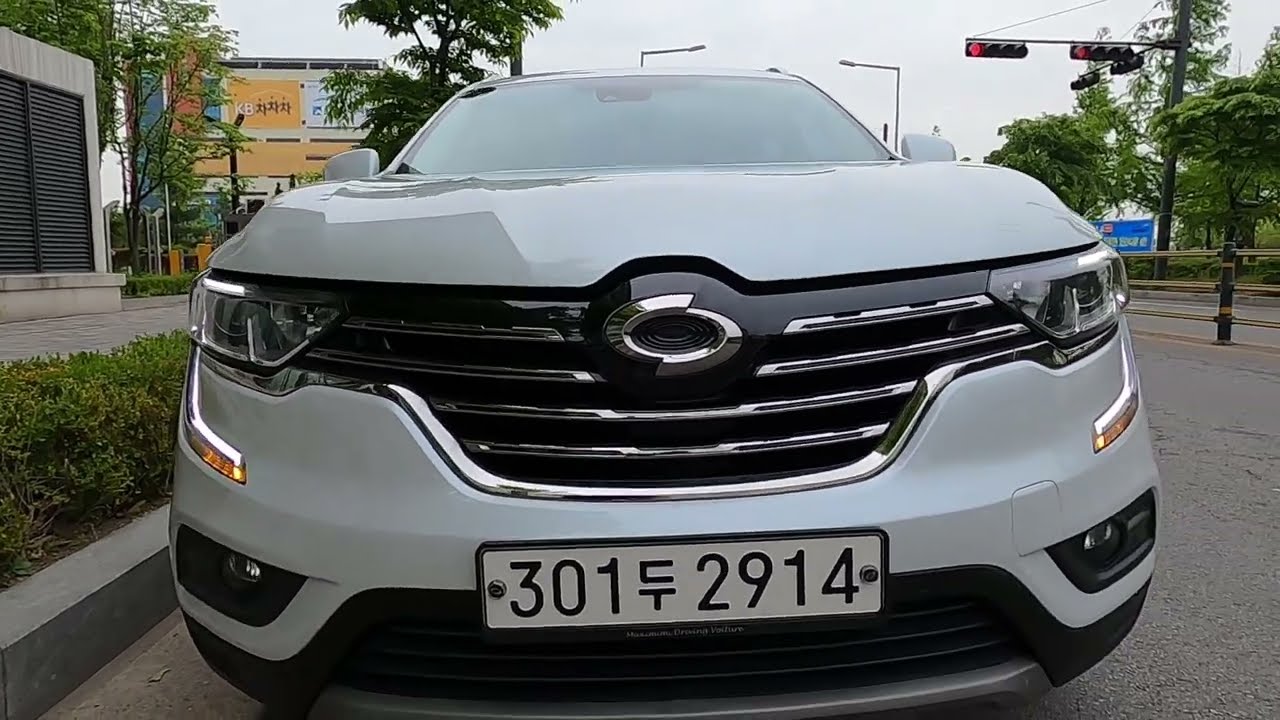In this close-up image of a white SUV taken in an outdoor setting, the vehicle's front grille, which is predominantly silver and black, occupies the majority of the frame. The SUV's distinctive silver logo is centered on the grille, just above a white, rectangular license plate. The plate features the numbers "301," the letters "CT" in a smaller font stacked on top of each other, and the numbers "2914," all in black. The plate is bordered in black and secured with bolts on both sides.

The image also shows the car's headlights, part of the hood, and the windshield, extending up to a portion of the roof. The SUV is parked on a gray asphalt surface. To the right of the vehicle, there's a metal fence, beyond which a roadway runs, marked by a double red traffic light on a nearby pole. In the background on the right, there are additional street lamps and trees lining the pavement.

To the left of the SUV, a low green hedge can be seen along a curb, with a sidewalk and buildings further in. An orange billboard with Asian characters is visible in the background, adding a splash of color to the scene. The setting provides a blend of urban and natural elements, framing the prominent vehicle at the image's center.